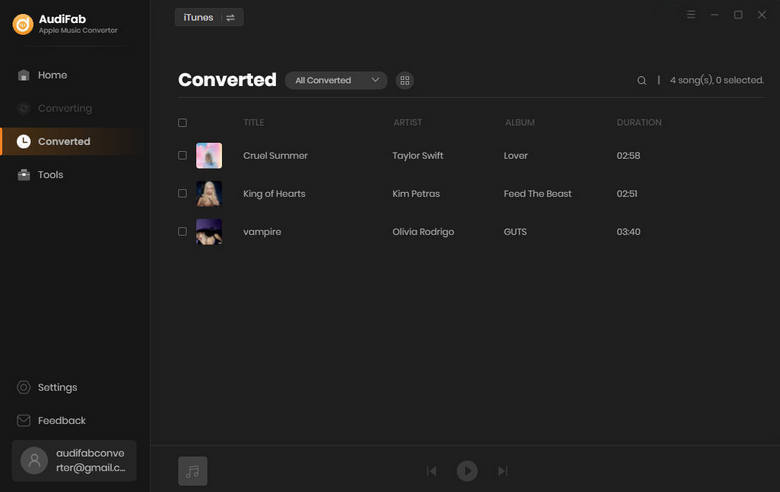In the image, we can see a software application with a sleek black background and white or gray lettering. The program is identified as "AudiFab Apple Music Converter," as indicated in the upper left corner. The left sidebar features several navigation options including Home, Converting, Converted, Tools, Settings, and Feedback, as well as a user icon displaying the username and email of the current user. The 'Converted' tab is currently highlighted in orange, indicating the active section.

On the right side of the interface, under the 'Converted' section, it shows that there are four songs listed with zero currently selected. The songs are organized in a detailed list format:

1. "Cruel Summer" by Taylor Swift from the album "Lover," duration 2 minutes and 58 seconds.
2. "King of Hearts" by Kim Petras from the album "Feed The Beast," duration 2 minutes and 51 seconds.
3. "Vampire" by Olivia Rodrigo from the album "Guts," duration 3 minutes and 40 seconds.

At the bottom of this section, there is a play button along with buttons that appear to be for fast-forwarding or skipping tracks. Additionally, an iTunes button is visible at the top of the interface, further indicating the software's functionality in converting Apple Music tracks, likely utilising iTunes. The organized layout and comprehensive list suggest a user-friendly and effective program for converting Apple Music tracks.